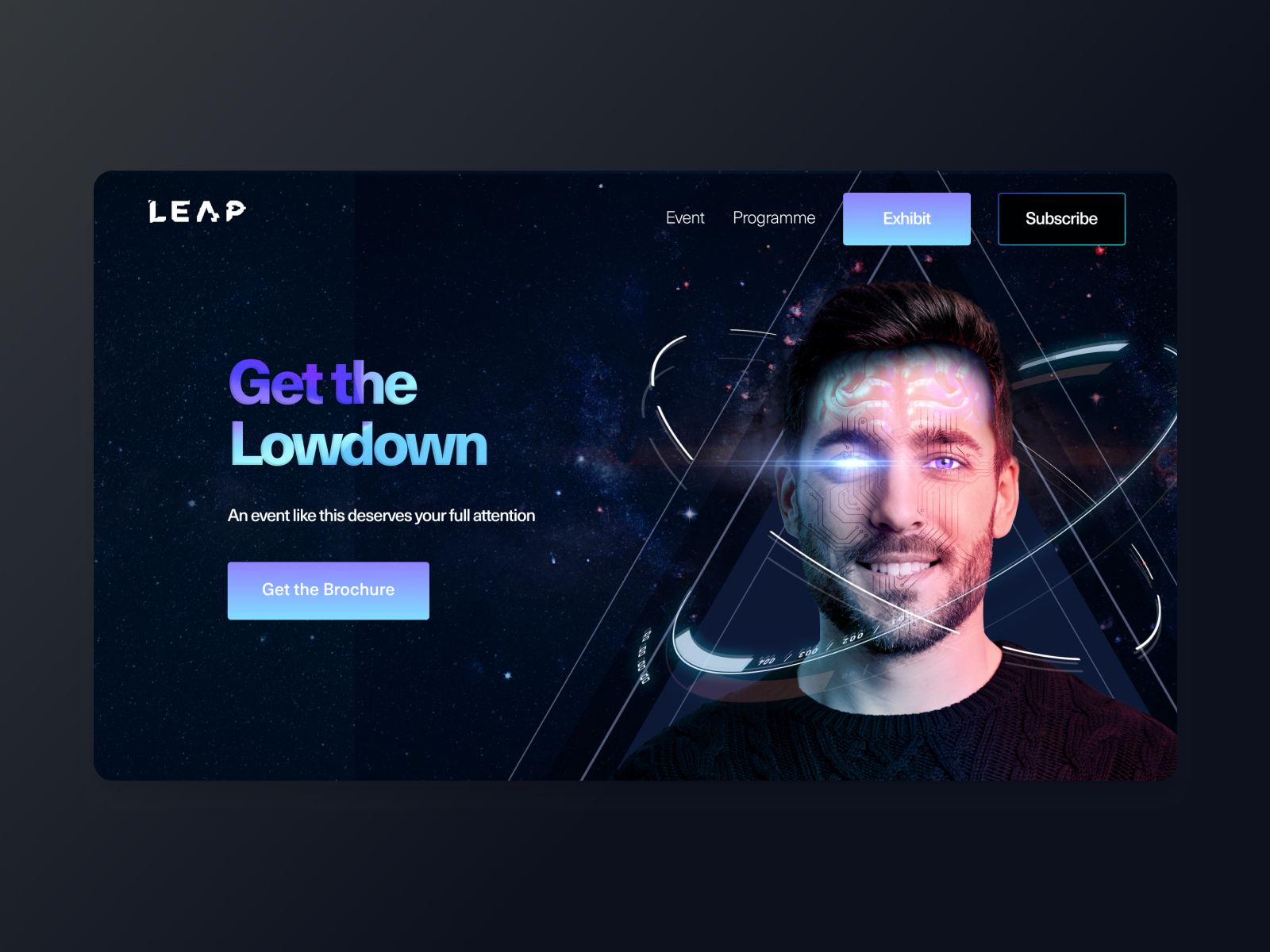This digital image features a screenshot of a website homepage set against a visually captivating background. The background showcases a gradient color transition from dark gray in the top left corner to dark bluish gray in the bottom right, portraying a starry night sky. 

The screenshot itself is a landscape-oriented rectangle with rounded corners. In the top left corner of the screenshot, the text “LEAP” appears in an all-caps, distressed white font, with the center bar of the 'A' missing, adding a stylized look. Following some negative space to the right, the words "EVENT" and "PROGRAMMED" (with double M's and an E at the end) appear in small white letters. 

Adjacent to this text are two interactive buttons. The first button has a gradient background blending light blue at the bottom into lavender at the top and features the white text "EXHIBIT" in its center. To its right, there is a black button with a gradient outline transitioning from bright blue at the bottom right to dark blue at the top left. This button has the word "SUBSCRIBE" in white text.

In the center left of the image, large text reads “GET THE LOWDOWN” in a gradient color that transitions from purple in the top left to bright blue in the bottom right. Below this prominent headline, a smaller line of white text reads: "An event like this deserves your full attention."

Situated below this, there is another button with a gradient color similar to the EXHIBIT button. This button bears the white text "GET THE BROCHURE" in its center.

This image combines a modern, visually engaging design with clear calls to action, making it an effective homepage layout for an event-focused website.